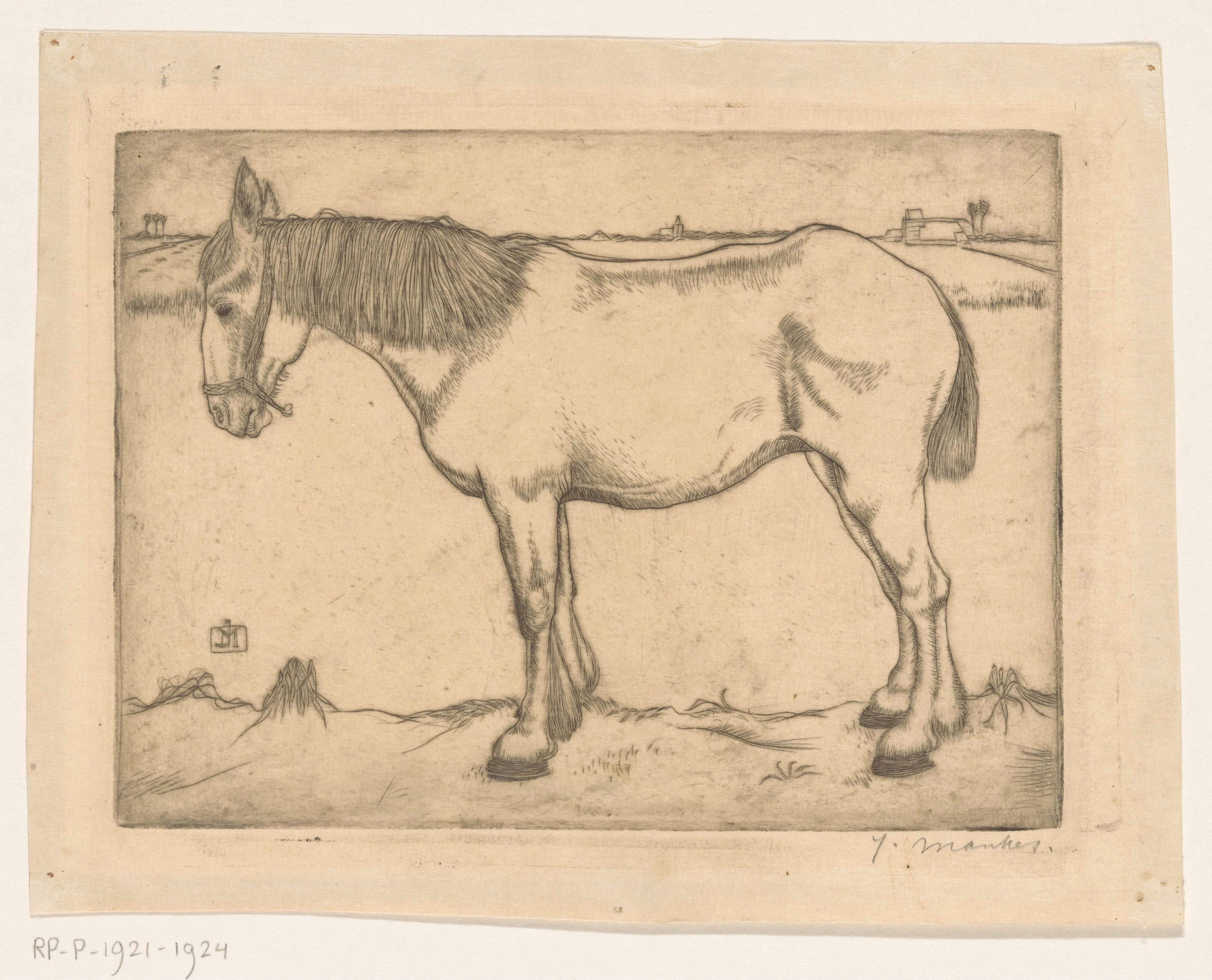This is a detailed black and white pencil drawing of a horse, presented on a thin, pinkish-beige parchment paper. The horse is the central focus, standing in a side profile view with remarkable detail in the depiction of its hair, muscles, and contours. It is wearing a halter and appears to be looking slightly downward. The ground beneath the horse is a mix of dirt and some emerging weeds, adding to the realistic yet somewhat barren setting. 

In the background, there is a field with a simple horizon line marked by a squiggly line, indicating distant trees and perhaps a very basic building or farmhouse, accompanied by what looks like a grain silo. This background creates a sense of depth and a Western, farmland ambiance. The drawing is enclosed within a rectangular pencil outline, further focusing attention on the detailed depiction of the horse.

At the bottom left corner, on the white border of the paper, there is a faint, possibly illegible signature which might read "T. Manker." Below this, there is a notation that says "R-P-P-1921-1924," adding a historical element to the piece. The overall composition is simple yet realistic, capturing a moment in a Western rural setting with a precise, skilled hand.